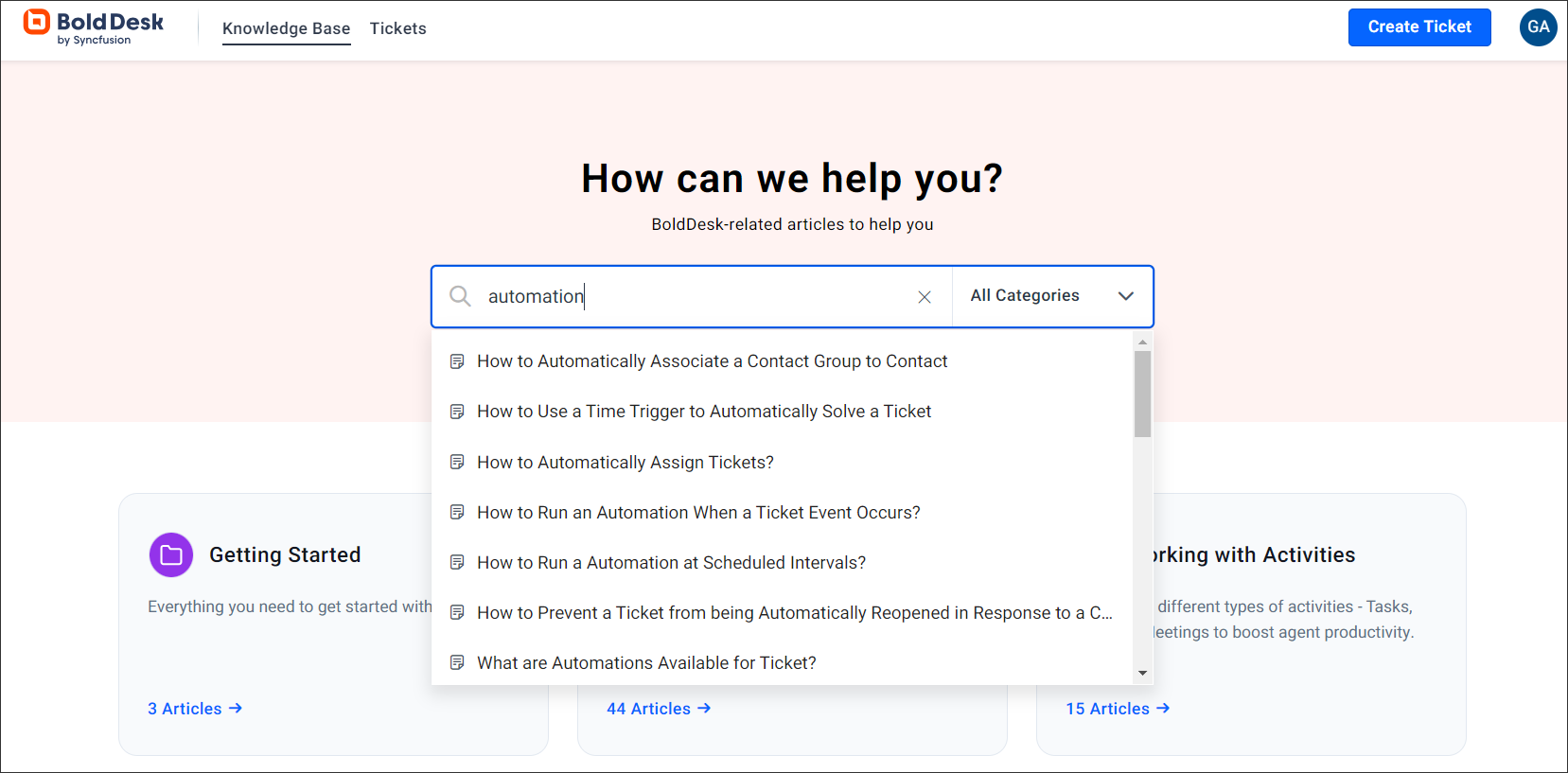The image is a detailed screenshot of the Bold Desk website by Syncfusion. Positioned at the top left is the Bold Desk logo. To its right are navigation options including "Knowledge Base" and "Tickets." On the far right, a prominent blue button labeled "Create Ticket" is visible, with "GA" immediately next to it.

Below this navigation bar, in a beige-colored section, a header reads "How can we help you? Bold Desk related articles to help you." This section includes a search box that contains the terms "Automation, All Categories." Below the search box, a list of search results is displayed, featuring titles such as "How to automatically associate a contact group to contact," "How to use a time trigger to automatically solve a ticket," "How to automatically assign tickets," "How to run an automation when a ticket event occurs," "How to run an automation at scheduled intervals," "How to prevent a ticket from being automatically reopened in response to a C...," and "What are automations available for a ticket?"

At the bottom of the page, there are links to additional articles, offering further resources for users navigating the site.